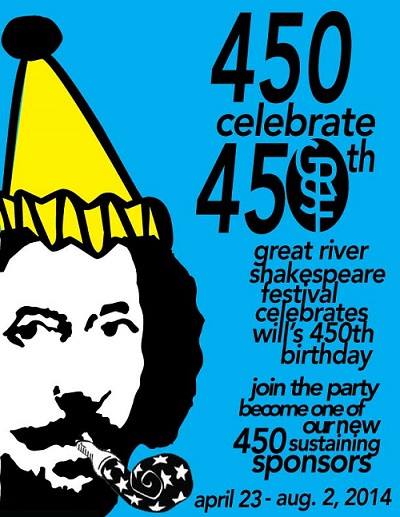This advertisement features the Great River Shakespeare Festival's celebration of William Shakespeare's 450th birthday. The event runs from April 23rd through August 2nd, 2014, and invites attendees to join the celebration and become one of the 450 sustaining sponsors. The background of the advertisement is light blue, with bold, black text prominently displaying "450 Celebrate 450th." The number "450" is significantly larger than the other text, and within the zero of the second "450," the acronym "GRSF" for Great River Shakespeare Festival can be seen. 

On the left side of the image, there is a clip art of William Shakespeare, depicted in black and white, wearing a festive yellow party hat with a black pom-pom on top. He has a party blower in his mouth, decorated with black and white stars. Shakespeare is portrayed with long hair, a mustache, and a beard. The advertisement’s colors predominantly include blue, black, white, and yellow.